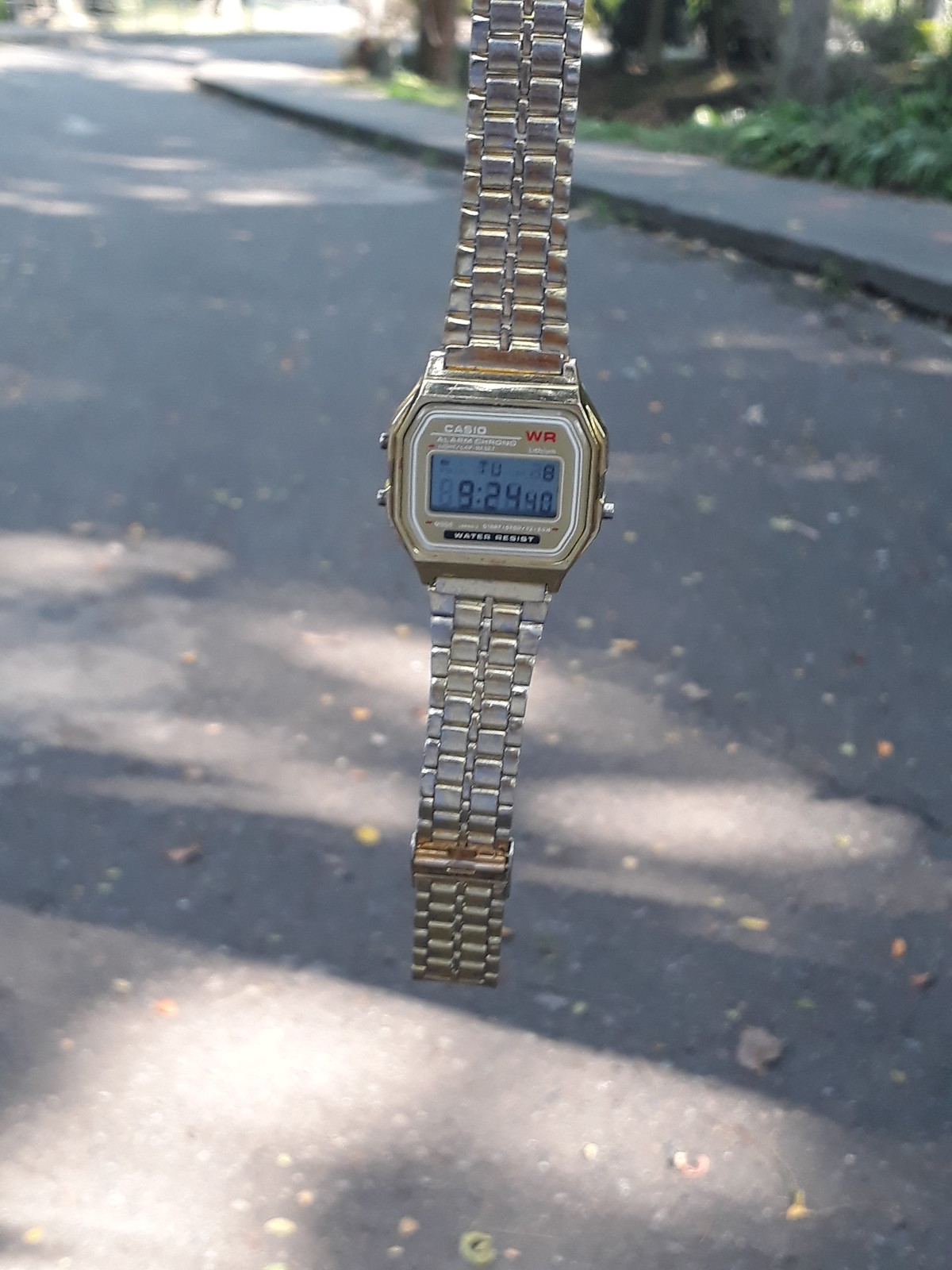This color photograph, taken outdoors in daylight, prominently features a stainless steel, digital Casio watch. The watch, centered in the image, appears to float mysteriously above a street with its top part out of frame, giving no indication whether it is being held or suspended by some unseen force. The digital screen of the watch displays the sequence "TU892440" and bears the inscriptions "Casio Alarm WR" and "Water Resistant." In the blurry background, a sidewalk lines the street, flanked by trees and lush greenery at their bases, creating a serene, natural setting.